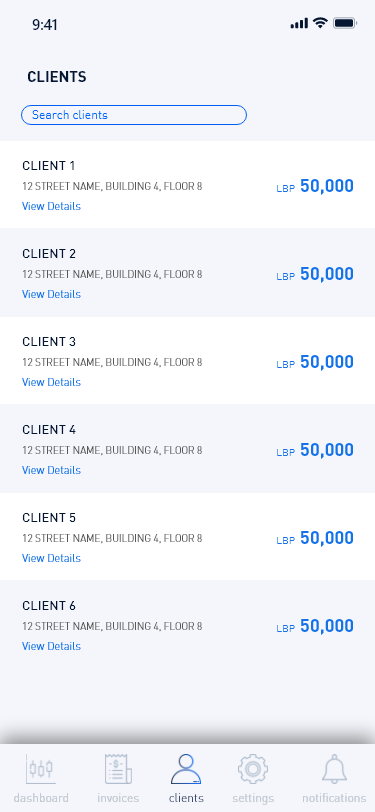In this image, we are looking at a smartphone screen displaying an app interface that lists clients. The phone's status bar is visible at the top of the screen, indicating its standard icons and time. Just below the status bar, the app header reads "Clients" with a search bar labeled "Search Clients." 

Beneath the search bar, there are six horizontal sections, each representing a different client. The sections are labeled sequentially: "Client 1, Client 2, Client 3," and so on, up to "Client 6." Each client entry includes the following details: 

- "12th Street Name, Building 4, Floor 8" – indicating the client's address.
- A clickable option labeled "View Details" for accessing more information about the client.
- An associated amount, "LBP 50,000," which could represent a fee, payment due, or another financial metric related to each client.

Interestingly, all six client entries share identical details regarding the address and financial amount, suggesting a template or repetitive data entry. The uniformity across all client listings implies that the specific customizable information is in some predetermined format or placeholder.